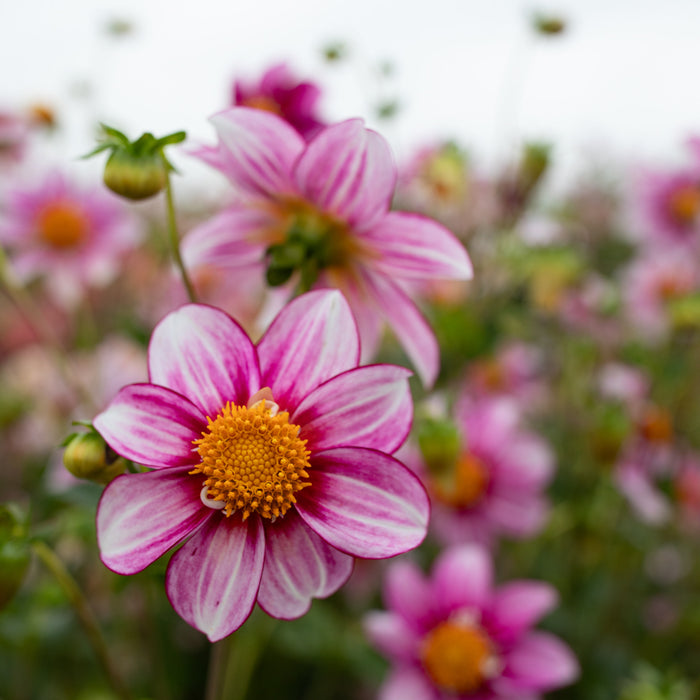The image captures a vibrant outdoor scene focusing on a stunning flower positioned off-center towards the bottom left. This prominently featured flower displays striking purple petals accentuated with delicate white highlights, surrounding a bright yellow center. Its green stalk is clearly visible, hinting at the flower still being attached. Behind it, a series of similar flowers add depth to the composition, though they progressively blur into a soft background. Additional stalks with unopened buds can also be noted. The background is a mix of greens with indistinct patches and features a white sky marred by what appear to be green dots, all under the bright daylight. The setting, likely a garden or a wildflower patch, adds a natural charm to the scene.